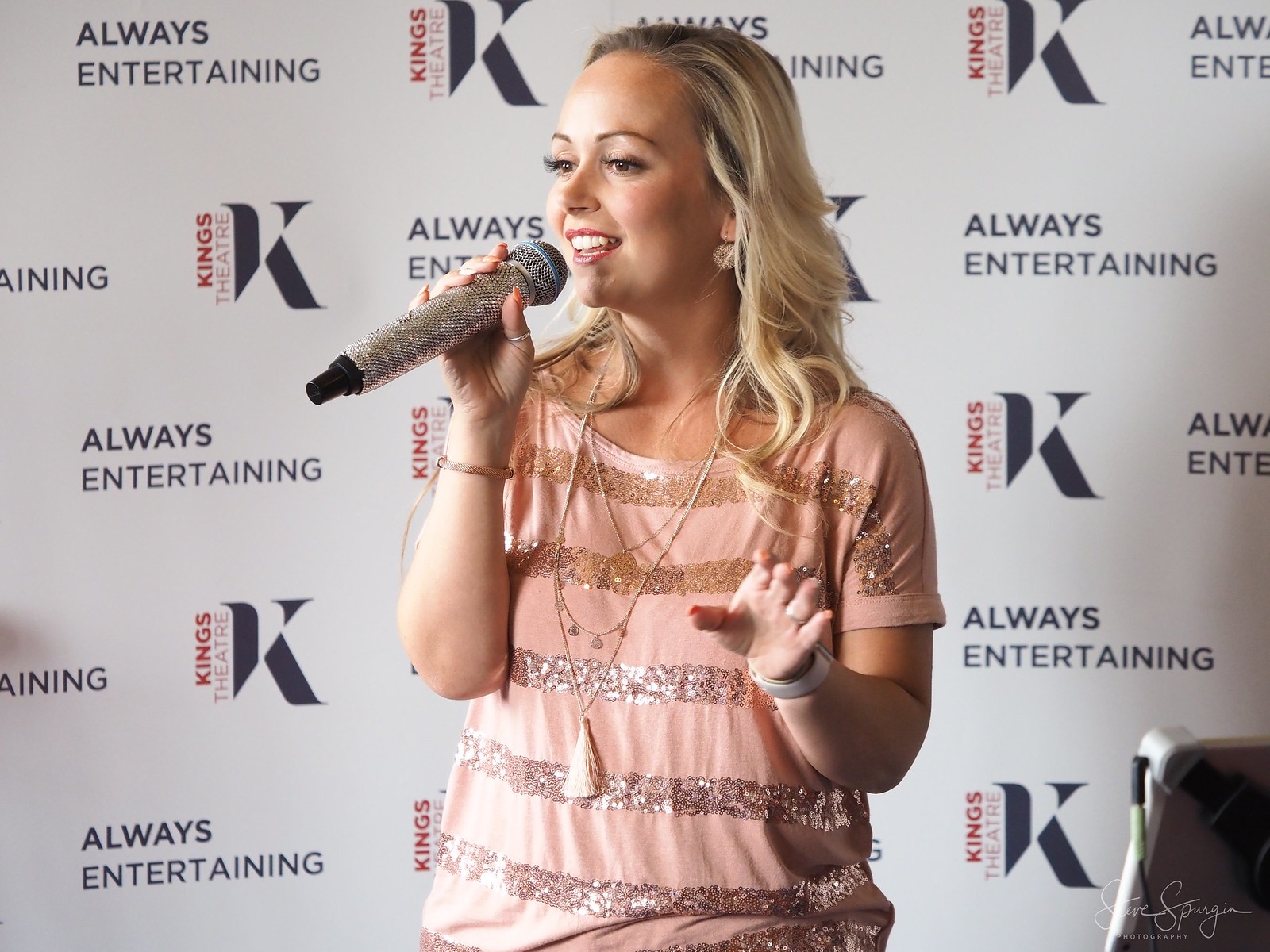This detailed photograph captures a dynamic moment of a woman with blonde hair speaking into a microphone. The backdrop is a white banner adorned with logos, including the phrases "Always Entertaining" and "King Theatre K." She appears to be hosting an event, perhaps as a comedian, and is fully engaged with her audience. She is wearing a distinctive, glittery pink striped top and accessorized with a white watch on her left wrist, a necklace, and gold dangling earrings. The microphone she holds in her right hand is also adorned with sparkles, adding to the glitzy ambiance. Her makeup is meticulously done, with coral lipstick and red-painted nails visible as she gestures expressively. The photograph, taken by Steve Spursia of Steve Spursia Photography, effectively captures the vibrant energy of the moment.